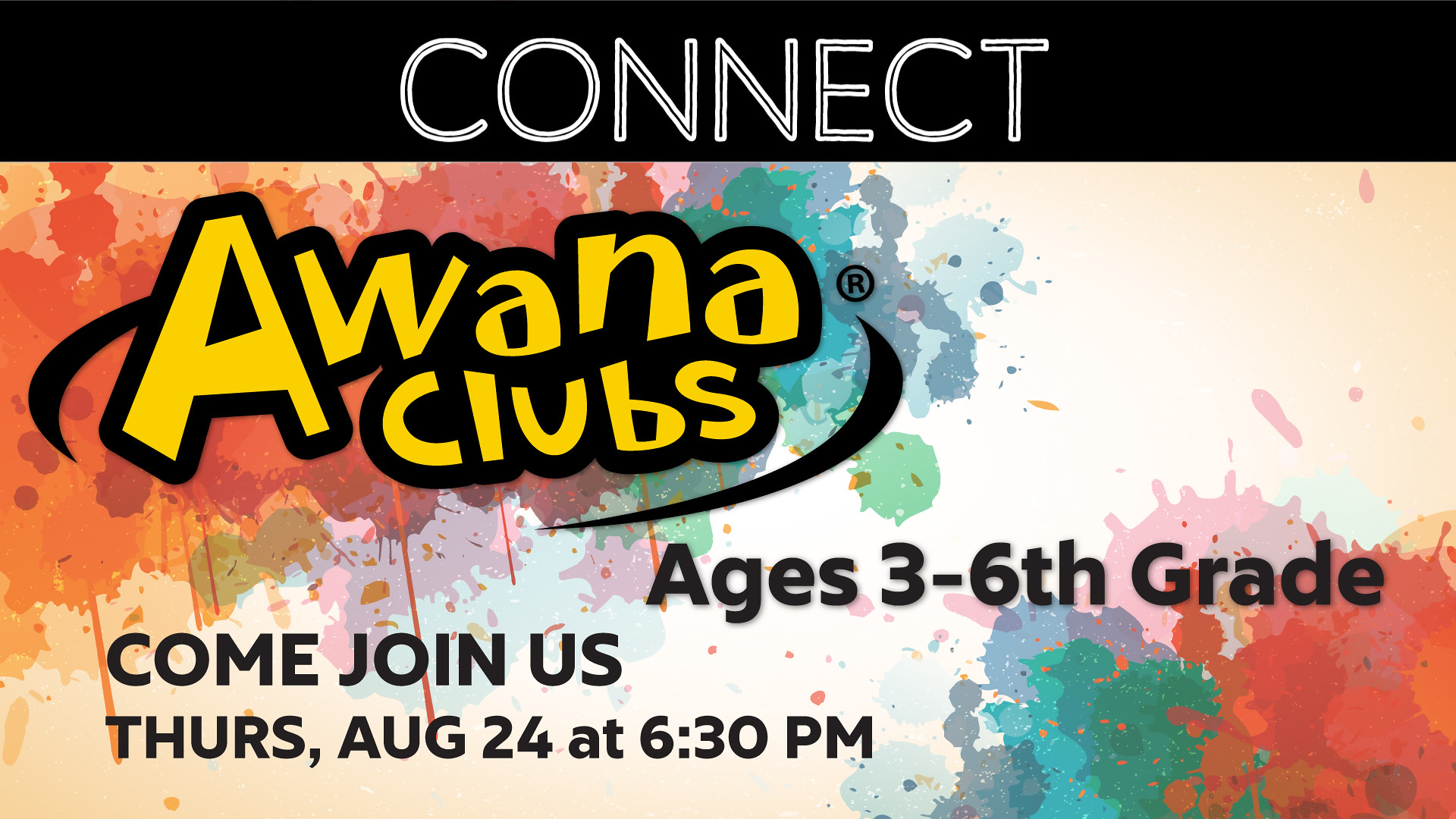The image is a horizontally aligned rectangular advertisement poster, presumably for social media or email use. It features a black strip bar at the top with bold white uppercase text that reads "CONNECT." Dominating the image is an abstract, colorful background resembling splattered watercolor paints. The upper left section showcases warm colors such as reds and oranges, while the middle features blues and purples. The lower right corner blends both warm and cool colors, including pink, green, blue, and light gray.

In the upper left corner, large bubble letters in bright yellow spell out "AWANA CLUBS," flanked by two curved black lines on each side. Midway down the right side, black text indicates "AGES 3-6th GRADE." The bottom left corner of the poster invites viewers with the message "COME JOIN US" in all-uppercase black letters, followed by "THURS, AUG 24th at 6.30pm." The overall design is vibrant and eye-catching, geared towards promoting a youth event organized by AWANA Clubs.